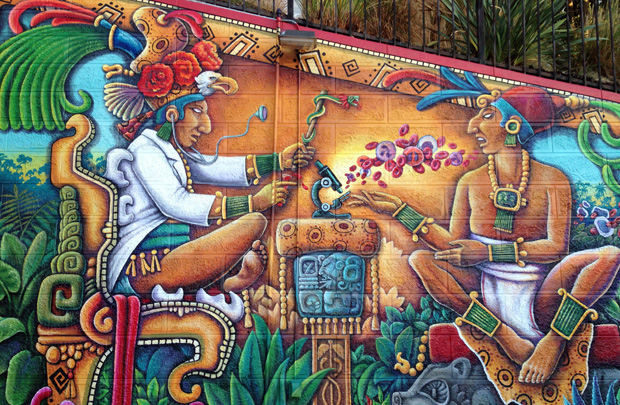This image showcases a vibrant mural painted on what appears to be the side of a brick or cement block building, possibly underneath a stairway with a black railing visible in the corner. The mural, rich in color, depicts an elaborate scene that merges elements of Egyptian and Native American art styles. Central to the composition are two figures seated across from each other at a table adorned with a microscope.

The figure on the left is a well-dressed individual wearing a white jacket and an ornate hat decorated with flowers. They are sitting cross-legged and have a stethoscope in their ears, intently examining the microscope. This person also holds a staff reminiscent of the Hippocratic Oath, featuring a snake coiled around it.

Opposing this figure, on the right, is a man who appears less formally dressed, wearing only a tunic and a striking yellow necklace with a gold pendant and green intarsia. He also adorns green wrist and ankle coverings, along with a red and blue feathered headpiece. This figure is depicted coughing, with red blood cells visibly emerging from his mouth, seemingly directed towards the microscope.

The mural intricately combines these symbolic elements, creating a scene that juxtaposes scientific inquiry with cultural and possibly mythological connotations.